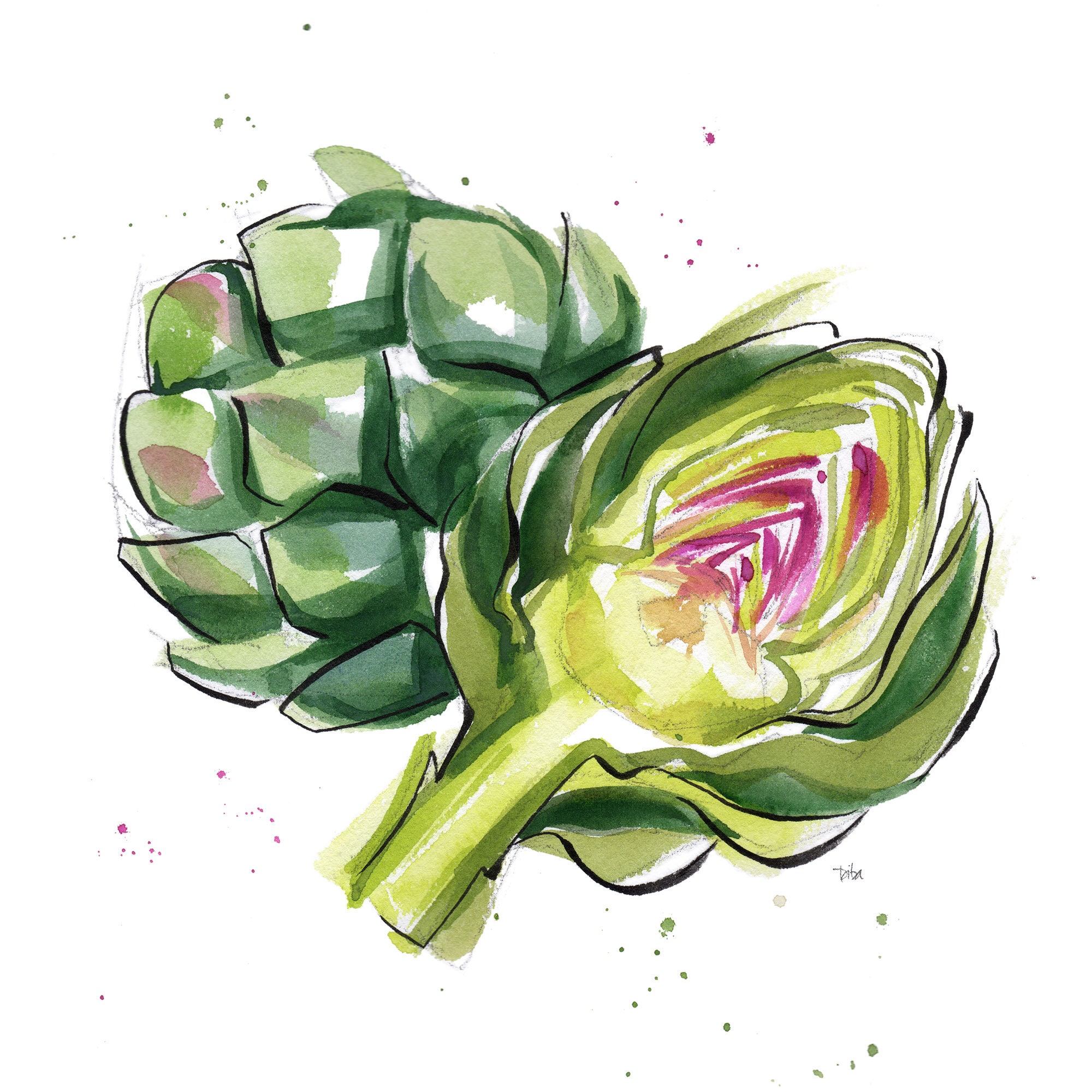This watercolor painting features two artichokes prominently displayed against a white background with no official border. The main artichoke is situated diagonally from the lower left-hand corner to the upper right-hand corner. It's sliced down the center, revealing a progression of darker green leaves on the outermost layer, which transition to lighter green, and finally to a pinkish-red interior. The intricate details include fine splatters of green around the main fixture, giving it an impressionistic feel. In the upper left-hand corner, the second artichoke is slightly behind the first, displaying more surface texture with its overlapping scales in shades of dark green, light green, and hints of pink. Beneath the slice of the front artichoke, there's a small signature in black text, likely the painter's autograph.